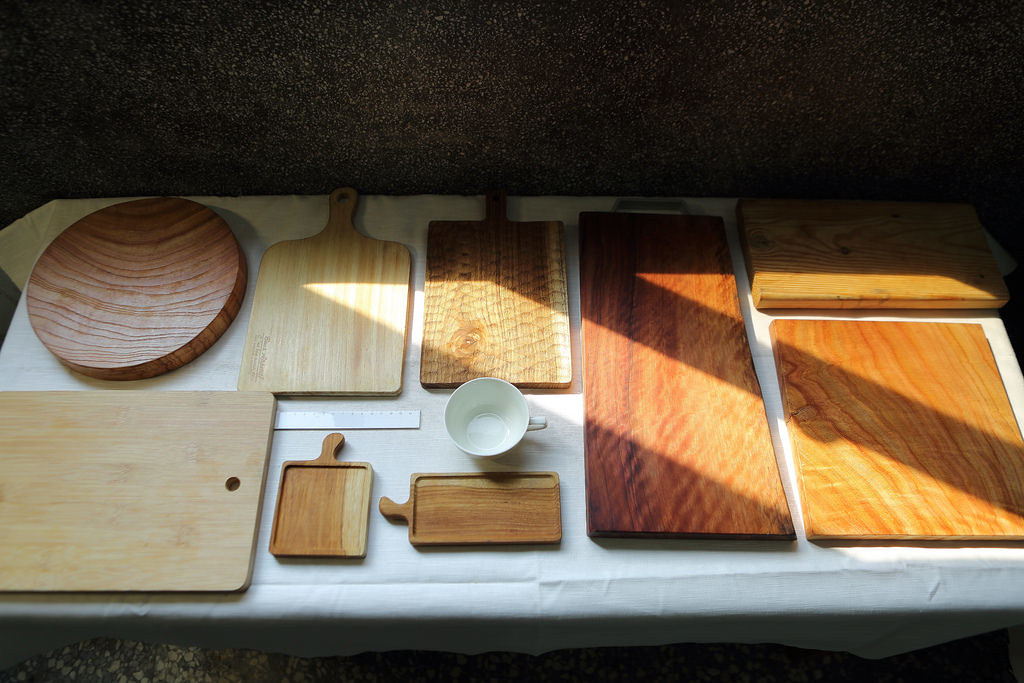This photograph showcases an array of wooden cutting boards of various shapes and sizes meticulously arranged on a table draped with a white tablecloth. The assortment includes a round cutting board, a square cutting board, and a rectangular cutting board. Additionally, there are two medium-sized cutting boards with handles, as well as two small cutting boards with curvy handles positioned at the bottom center of the image. These boards, exhibiting different shades and grain patterns of wood, are complemented by a white teacup and a ruler placed strategically in the center to indicate scale. The scene is bathed in sunlight streaming through an unseen window, casting a natural light on some of the items. In the backdrop, a wall with a dark speckled color adds contrast, while a unique tiled floor resembling smashed rocks completes the setting.